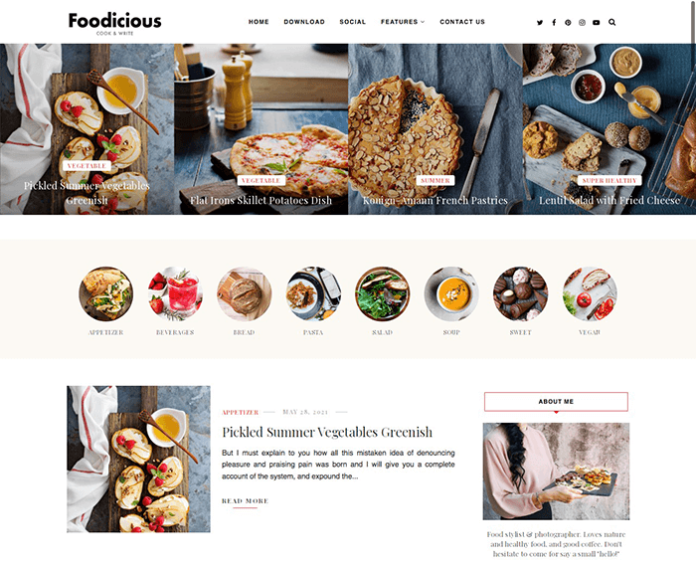The image depicts a vibrant and detailed food blog page titled "Fooditious." At the top of the page is the title "Fooditious," followed by the tagline "Cookin' Cookin'." This suggests that the page focuses on sharing recipes and cooking techniques. To the right of the title, there's a navigation menu with options such as Home, Download, Social Features (with a drop-down box), and Contact Us. Social media icons for Twitter, Facebook, YouTube, and other platforms are also visible, indicating ways to connect and engage with the content.

The main section of the page showcases a series of four mouth-watering food pictures, each representing a unique recipe. The first picture features a recipe for pickled summer vegetables displayed on a rustic wooden palette, accompanied by what looks like buttery toast with cheeses and fruit. The second image showcases a hearty skillet potato dish that resembles a pizza. The third photo presents French pastries, ideal for a warm summer day. The final image is of a healthy lentil salad topped with fried cheese, offering a nutritious option for health-conscious readers.

Beneath these images, a row of categories with icons and images allows users to explore different types of recipes, including Appetizers, Beverages, Bread, Paninis, Salads, Soups, Sweets, and Vegetables. To the right, an 'About Me' section introduces the food stylist behind these delectable dishes, providing insight into her culinary journey and expertise.

On the left, the current highlighted recipe is the pickled summer vegetable appetizer. The description hints at initial mistakes made during the preparation process and reassures readers that following the detailed directions will lead to a successful and tasty outcome. The page combines an appealing mix of visual delight and practical cooking advice, making it a comprehensive resource for food enthusiasts.